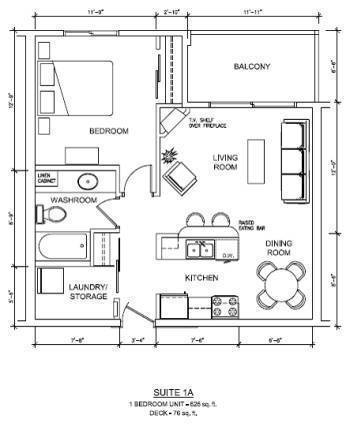This is a meticulously drawn floor plan of a one-bedroom unit labeled as "Suite 1A," rendered on a white sheet of paper. The layout begins at the bottom of the page with the front door. Immediately to the right of the entrance is a compact kitchen featuring a refrigerator, a stove, and a countertop equipped with sinks. Adjacent to the kitchen is a cozy dining area. This space seamlessly transitions into a spacious living room, complete with a couch, coffee table, television, and an armchair. 

At the top of the drawing, a large balcony extends across, adding an inviting outdoor space. Moving to the left side of the floor plan, starting from the bottom, there is a small room dedicated to laundry and storage, indicated by a black box. Next to this is the bathroom, which contains a toilet, a sink with a countertop, and a cabinet for additional storage.

Finally, the bedroom occupies the leftmost section of the layout. It is generously sized and includes a bed, flanked by what appear to be four rectangular nightstands, and features a smaller rectangle against the wall likely representing a dresser. This thoughtfully arranged floor plan ensures a blend of functional living spaces and comfort in a well-proportioned design.